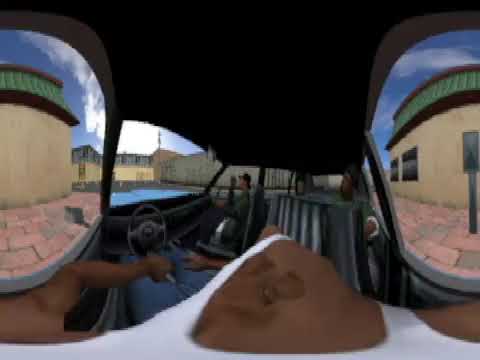The image captures a 360-degree panoramic view from within a vehicle cabin characterized by significant distortions, making its true shape challenging to ascertain. The interior bears similarities to both a car and a boat, with defining features including a brown dashboard and a prominent steering wheel situated centrally. The cabin, enveloped by expansive glass windows, is illuminated by natural light, hinting at its potential to be a boat cabin or a car interior. There are two visible men in green shirts occupying black leather or pleather seats, possibly captain's chairs, which denotes a sense of structured seating like in a cockpit. Additionally, a person with a tan shirt appears to be present, evidenced by visible arms. The exterior scene reveals a blue expanse beneath the vehicle—likely water—bordered by walkways composed of pink bricks or massive blocks, extending alongside tan cinder block walls punctuated by windows. The background showcases a lineup of buildings, adding further context to the setting. The low-resolution nature of the image indicates it may have been captured using VR, contributing to the misshapen and blurry visual elements.